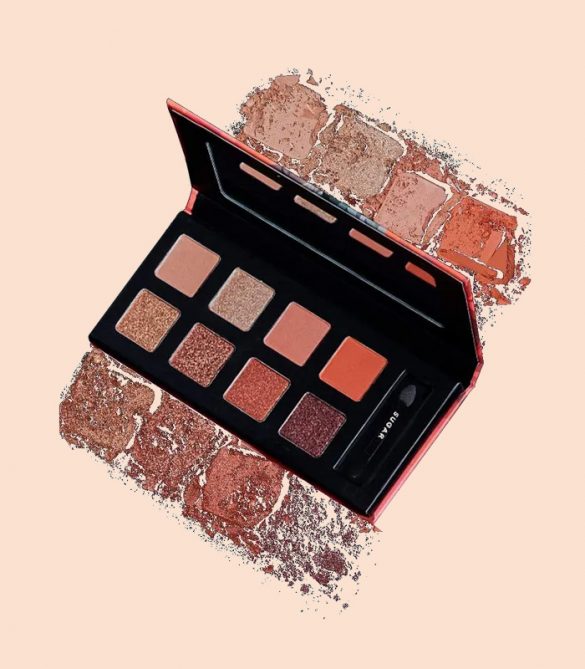The image depicts an advertisement for a makeup palette, prominently featuring the word "sugar." The palette contains eight eyeshadows with a mix of five shimmery shades and three matte ones, mainly in warm rosy pinks, browns, peaches, reds, and a touch of purple and gold. The makeup case is open at a 90-degree angle, revealing its sleek black interior with a small applicator tucked on the right side. The compact also includes a mirror reflecting part of the palette, and is set against a light pinkish-tan background, mimicking the look of skin. The image is accented by sample makeup crushed and spread around it, showcasing the shimmery textures and diverse hues.